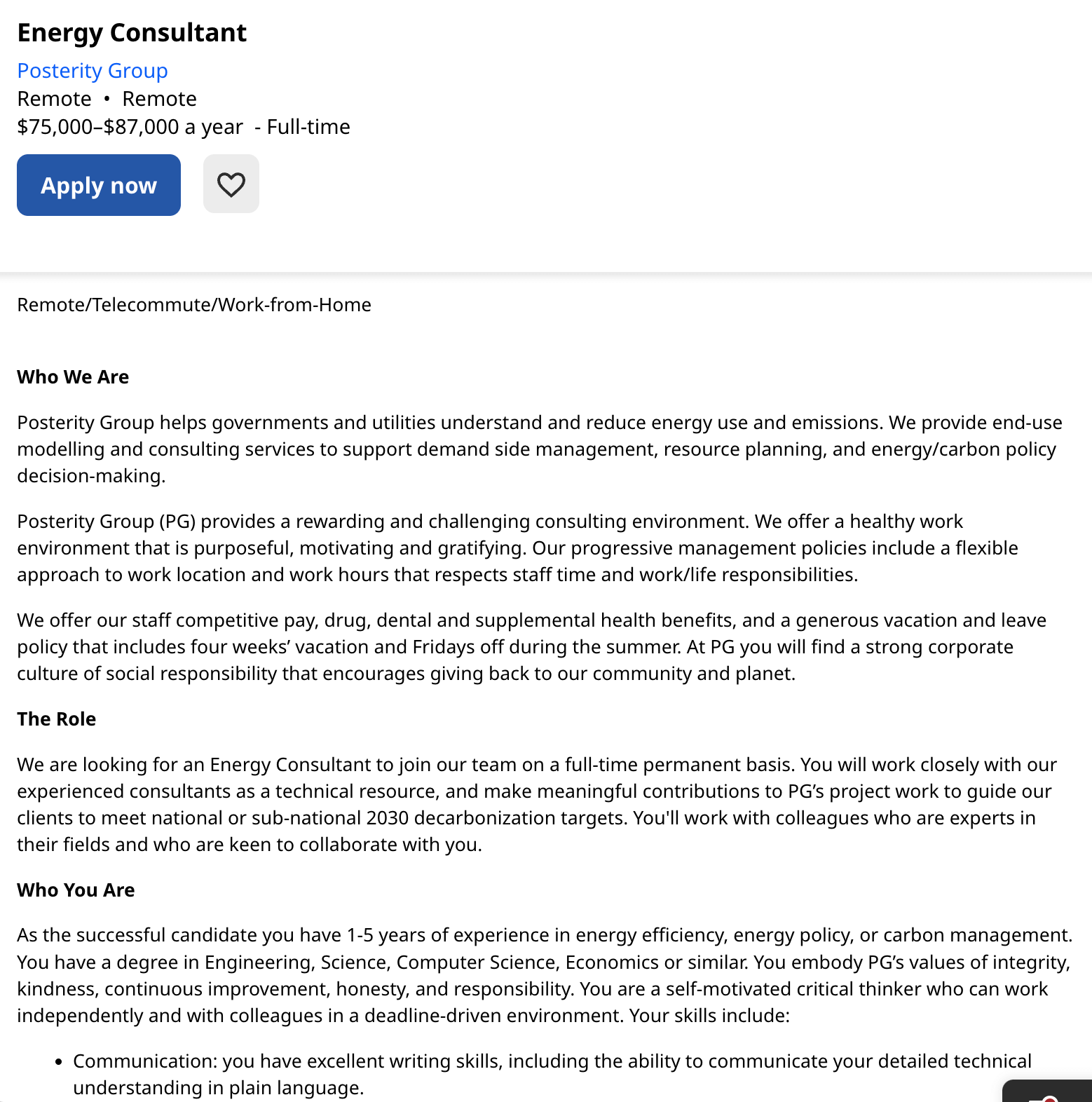**Detailed Job Posting for Energy Consultant at Prosperity Group**

---

**Position:** Energy Consultant   
**Company:** Prosperity Group   
**Location:** Remote, Work from Home   
**Employment Type:** Full-time   
**Salary Range:** $75,000 to $87,000 per year   

---

**Apply Now** | ♥ Save Job   

---

**About Us**

**Prosperity Group (PG)**: We assist government agencies and utility companies in understanding and decreasing energy use and emissions. Our services include end-use modeling and consulting aimed at supporting demand-side management, resource planning, and energy carbon policy decision-making.

**Our Work Environment**

At PG, we foster a rewarding and challenging consulting environment. We pride ourselves on maintaining a healthy workplace that is both purposeful and motivating. Our progressive management policies promote flexibility in work location and hours, respecting our staff's time and work-life balance.

**Benefits and Compensation**

- **Competitive Pay:** Annual salary ranging from $75,000 to $87,000.
- **Comprehensive Health Benefits:** Includes drug, dental, and supplemental health care.
- **Generous Leave Policy:** Four weeks of vacation and Fridays off during the summer.

**Our Culture**

Prosperity Group emphasizes social responsibility within our corporate culture, ensuring that our work not only benefits our clients but also contributes positively to society.

Join a team where you can make a meaningful impact on energy use and emission reductions while enjoying a flexible, supportive work environment.

---

[Apply Now Button]

[Save Job Button]

---

**Remote Work, Telecommute, Work from Home**